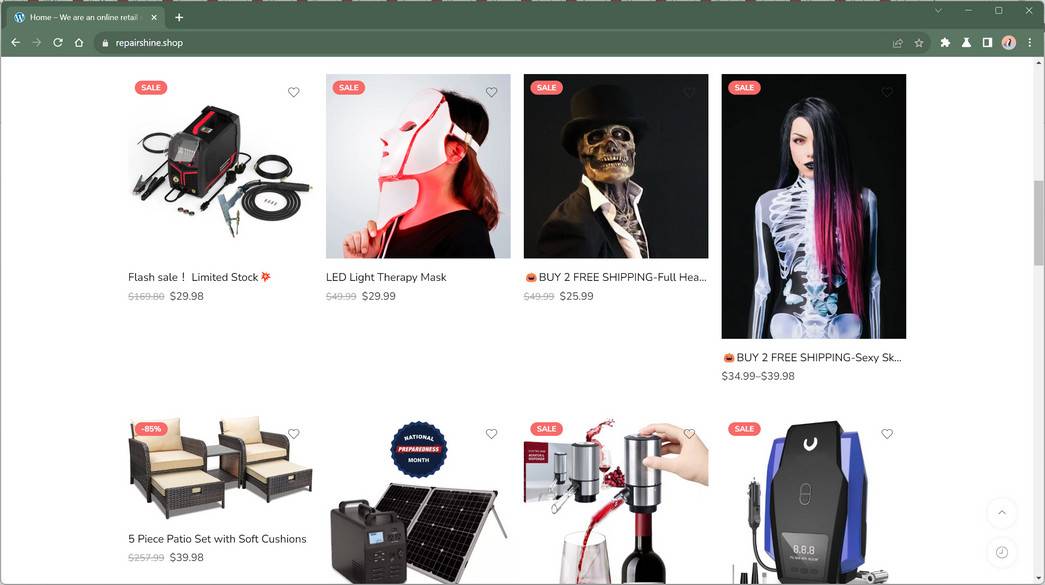This image appears to be a screenshot of an online shopping website, "RepairShine.shop," featuring a layout of items available for purchase. The upper left corner of the screenshot shows an open tab labeled "Home" next to the site's logo and navigation buttons, including forward, back, and refresh. The central part of the page displays a grid of eight items for sale. 

The top row includes:
1. A battery-type charger.
2. An LED light therapy mask.
3. A Halloween mask.
4. A Halloween costume.

The bottom row features:
1. Two couches, each equipped with a pull-out leg rest.

The page layout and product images suggest a diverse selection of items aimed at a broad range of customer needs, from electronics to seasonal costumes and home furnishings.